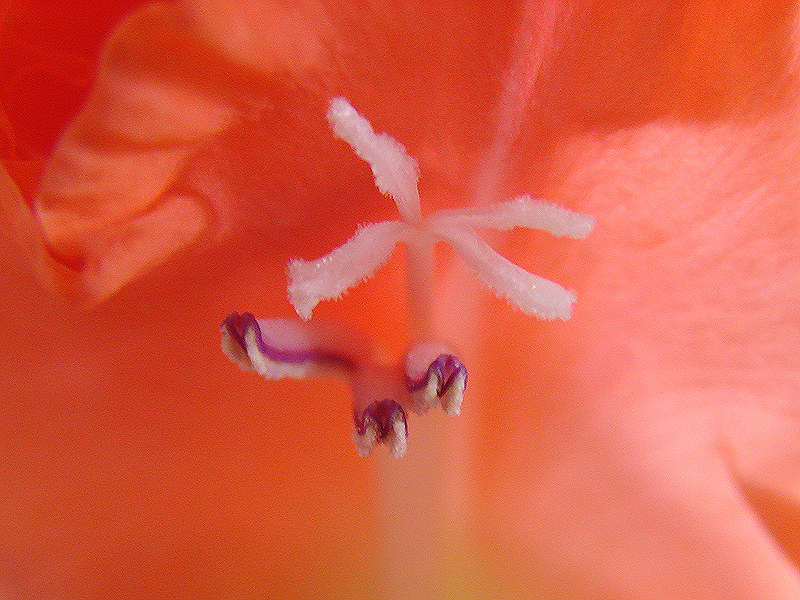This photograph captures an extreme close-up of the center of a flower, likely a rose, characterized by its vibrant pink petals that form an out-of-focus backdrop. Dominating the scene is a fuzzy, white central stem, possibly the flower's stamen, which extends into four delicate, tentacle-like filaments. Adjacent to this central structure are three additional appendages adorned with a striking purple stripe running along their lengths, seamlessly transitioning to soft, white strands at their tips. These structures appear pink at their base, contributing to the overall texture and complexity of the image. The photograph's intense magnification highlights intricate details not commonly visible to the naked eye, portraying a mesmerizing and almost otherworldly view of floral anatomy.